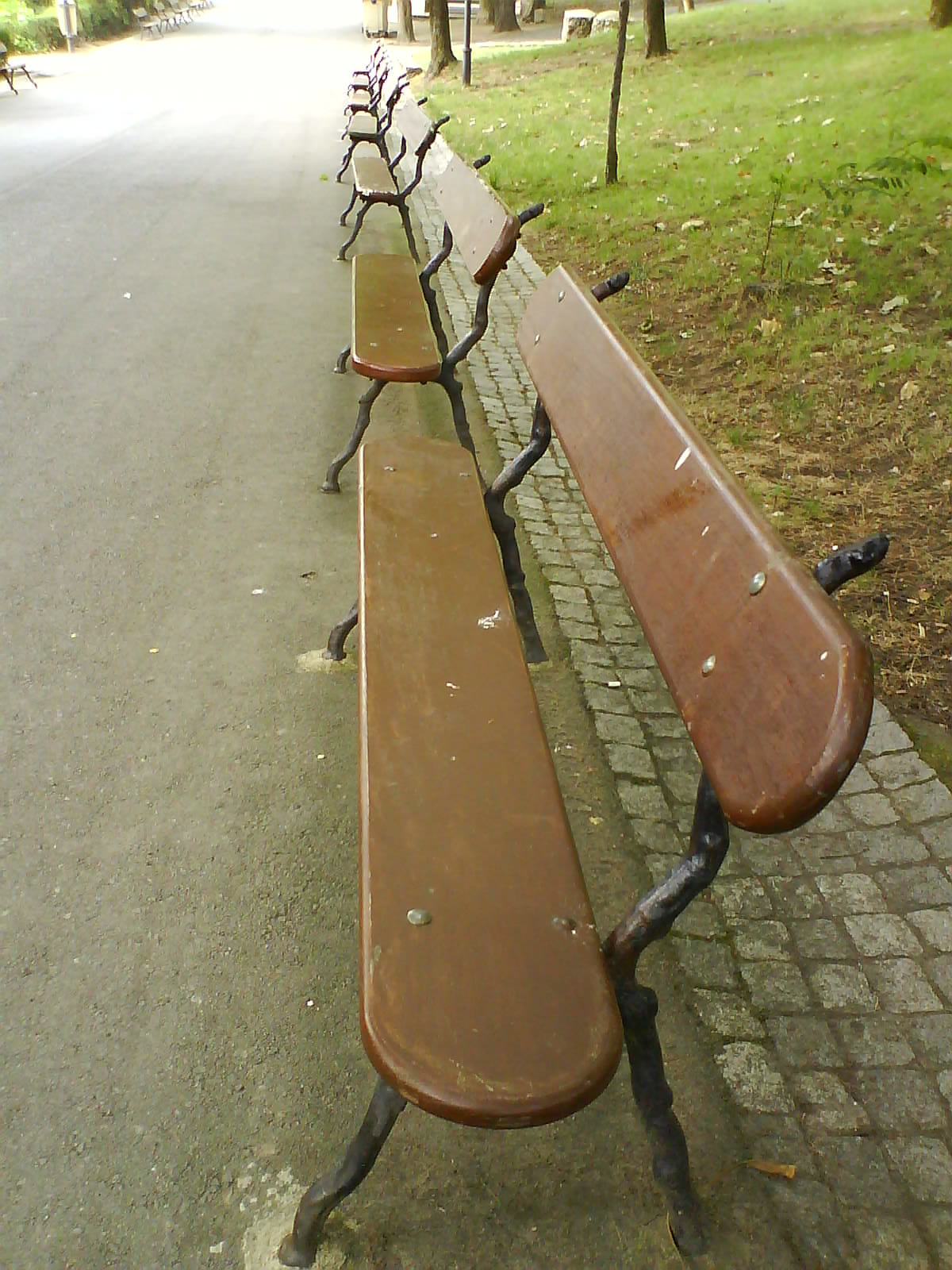In this outdoor daytime photograph, the composition centers around a row of park benches, which extend vertically through the image's center. Each bench features a long, narrow wooden seat and backrest, both in brown, supported by black wrought iron frames with a round design. The benches, numbering six or seven, appear in a straight line, with visible variations such as dirt marks and white stains on some.

To the left of the benches is a tan walking path or road, followed by a gray brick sidewalk bordered by a cobblestone gutter. Beyond the cobblestone sidewalk lies a green field with patches of brown grass and scattered leaves. In the background, the bases of a few tree trunks are visible, though their foliage remains out of frame. The serene park setting is unmarred by any text or printing, emphasizing the well-maintained yet slightly weathered benches and the natural surroundings.